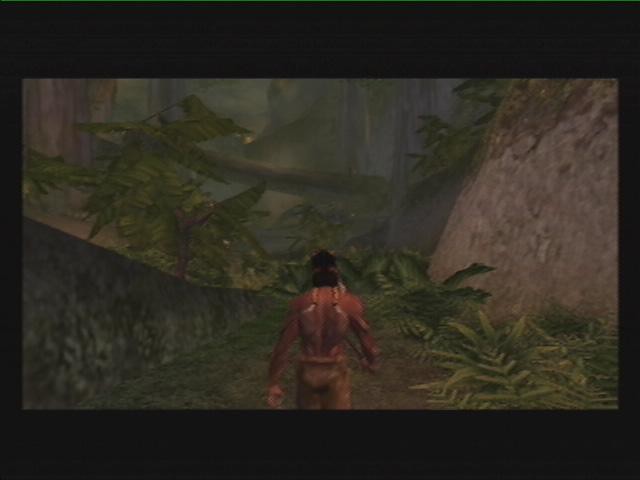This screenshot, likely from a video game, features a detailed jungle scene framed by a black border. The top border is notably thick, accounting for around 15% of the image's height, while thinner borders run along the bottom and sides. The scene is wider than it is tall, enhancing the wide-angle effect. Dominating the environment are ferns and lush foliage that cover the ground and climb up the left side and into the corners of the frame. On the right, a towering rock face with ferns and boulders adds a rugged texture to the background. The atmosphere is dark and smoky, suggesting either nighttime or heavy mist.

In the center of the frame stands a warrior, depicted from his mid-thigh up in a third-person perspective. He is reminiscent of characters from the game Turok, with darker skin, medium-length black hair, and a red headband. The warrior wears minimal clothing, possibly a loincloth or fur, revealing his bare torso. He also seems to be holding a sword or similar weapon. The right side of the frame shows additional leaves of varying shades of green, some with yellow specks, and further in the distance are more trees, casting shadows and deepening the sense of dense jungle foliage.